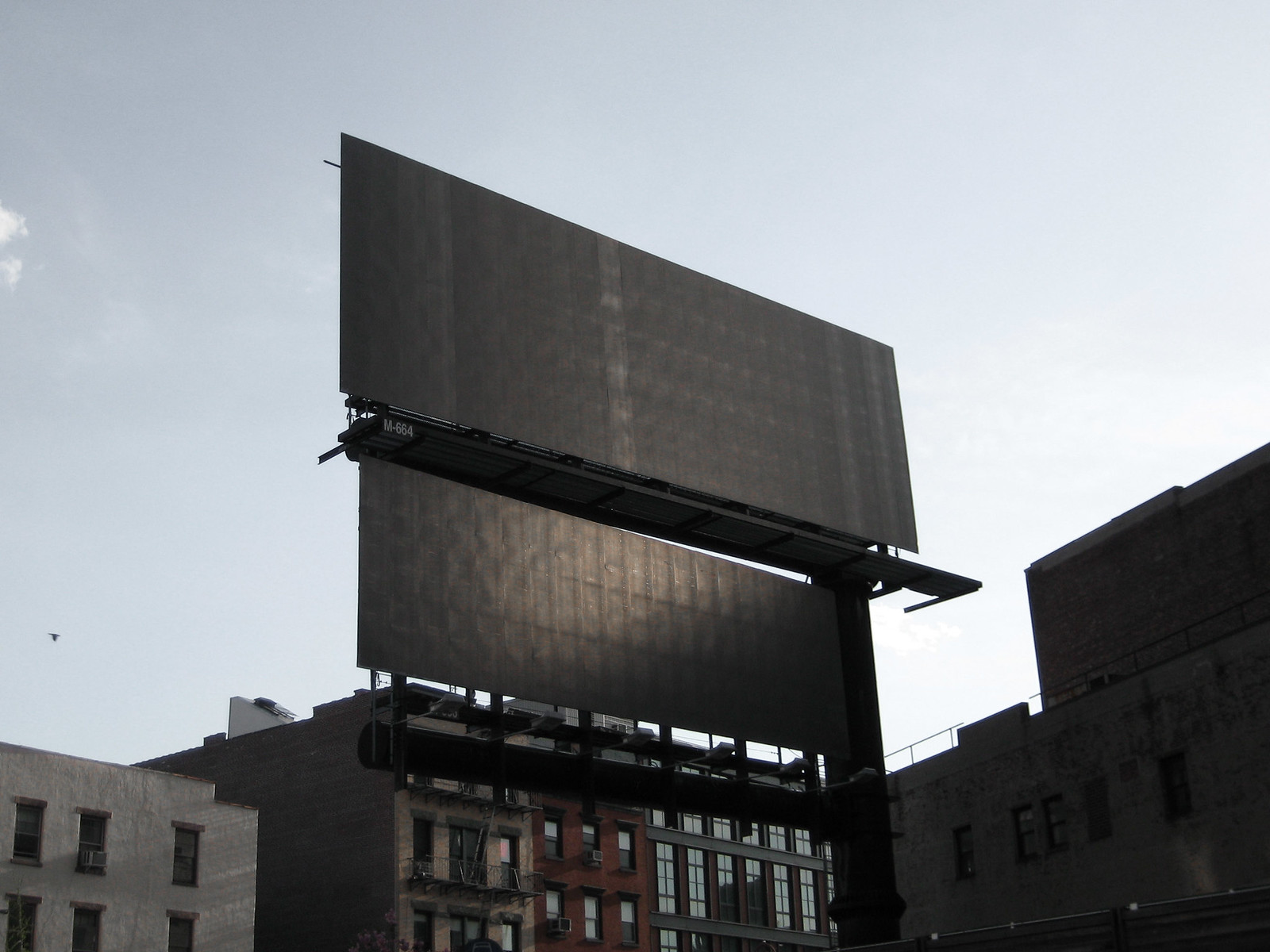A bustling urban scene captured during the transition between day and night, the photograph showcases a mixture of downtown commercial buildings and residential apartment complexes. The buildings dominate the frame, their mostly beige exteriors interspersed with one prominent structure painted in a deep reddish-orange hue, leaning more towards red. The sky above is a light to medium blue, suggesting the moments of either sunrise or sunset, as the overall ambiance is dim with minimal direct sunlight. Wisps of white, fluffy clouds sporadically dot the horizon, adding texture to the otherwise clear sky. In the midst of this urban landscape, two billboards stand out, both entirely black, possibly indicating that any previous advertisements or images have been painted over or obscured. The combination of architectural elements and slight twilight casts a serene yet mysterious mood over the cityscape.